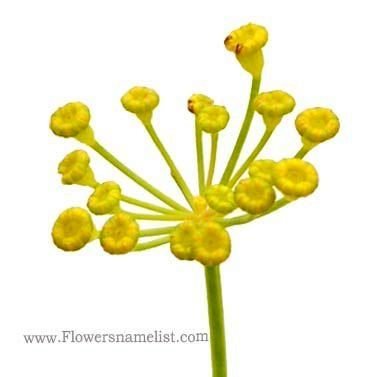The image appears to be a computer-generated portrayal of a botanical subject, featuring a tall, green stem that branches out into numerous smaller stems, each bearing a small, round, bright yellow flower. The flowers exhibit a bell-like shape and are predominantly yellow, with a few petals tinged red. Each flower has six sections or petals, reminiscent of an inner tube raft, converging into a cone that joins with the stem. Approximately 18 to 20 flowers can be observed emerging from the lime-green, almost yellowish-green stems, all set against a stark white background. An inscription in the lower left corner reads "www.flowersnamelist.com," suggesting the image might be sourced from an online flower database for educational purposes or botanical identification.